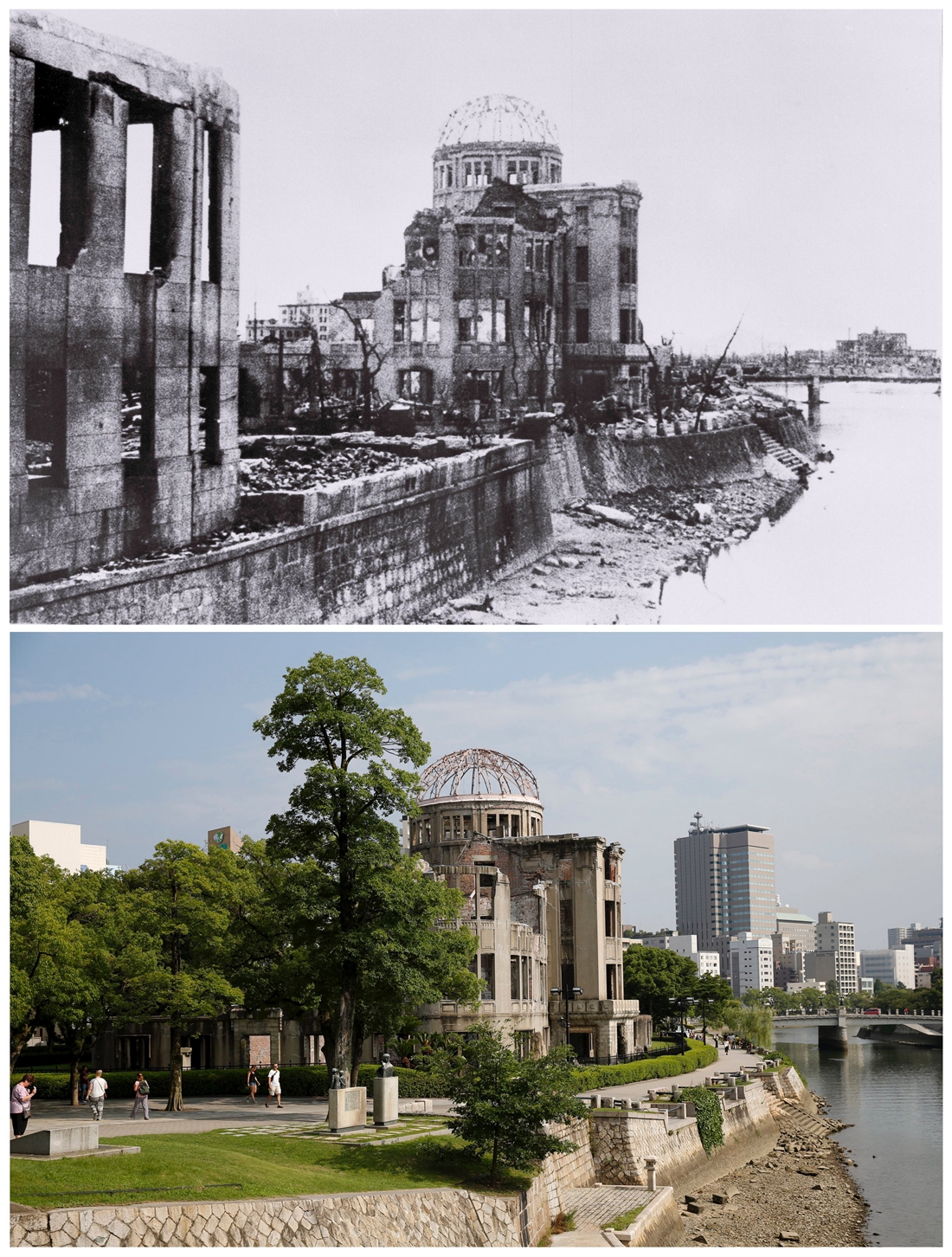The image is a juxtaposition of two photographs showcasing the iconic Hiroshima Peace Memorial, also known as the Atomic Bomb Dome. The image is split into two halves, with the top half presenting a stark black-and-white photograph from shortly after the Hiroshima bombing, while the bottom half displays a modern, full-color photograph of the same site.

In the top half of the image, the building appears severely damaged, with crumbled walls and blown-out windows. The dome atop the structure is intact but charred, emphasizing the extent of devastation. Surrounding the structure are remnants of other buildings and trees that have been burned, and the shoreline along a nearby river is lined with large stone walls and stairs leading down to the water. The background is desolate, highlighting the dramatic contrast with today's view.

The bottom half shows a contemporary, vibrant scene where the building, though still worn and broken, stands as a preserved ruin—a memorial to the events of the past. The perspective is nearly identical to the historical photograph, showcasing the stone walls and stairs leading down to the water, which have remained unchanged. Modern high-rise buildings and a city skyline rise in the distance. The area has been meticulously maintained with lush trees and a picturesque promenade, along with two small bronze statues placed in the park area near the building. Overall, this half of the image reflects the growth and rebuilding of Hiroshima while preserving the memory of its history.